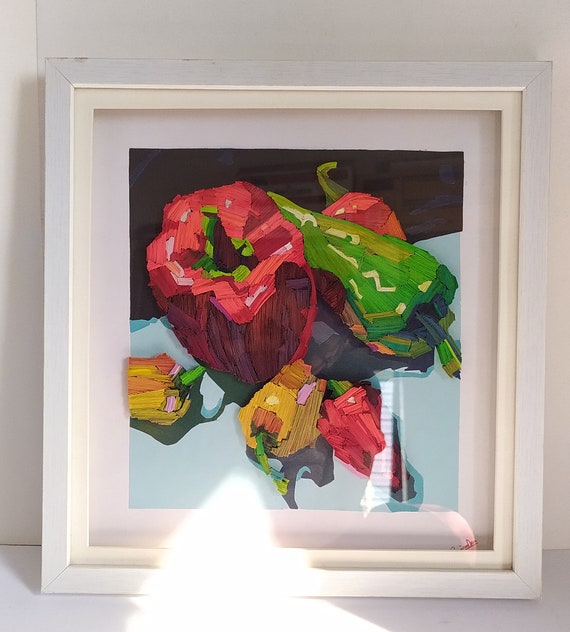This photograph captures a framed piece of artwork leaning against a light gray or beige wall. The frame itself and the matting inside are both white, and the frame rests on a white ledge. A prominent triangular glare is visible, extending from the center bottom of the photo across the frame. The painting, done in a cubist or abstract style, features a variety of peppers with geometric, angular forms, rather than smooth, rounded edges. The central figures include a large red bell pepper, a green jalapeño pepper, and several smaller red and yellow peppers, all depicted with green stems. The background of the painting transitions from black at the top to white at the bottom, creating a stark contrast where the peppers appear to be placed on a white surface. Notably, there is a red signature in the lower right corner of the painting, partially obscured by the frame.